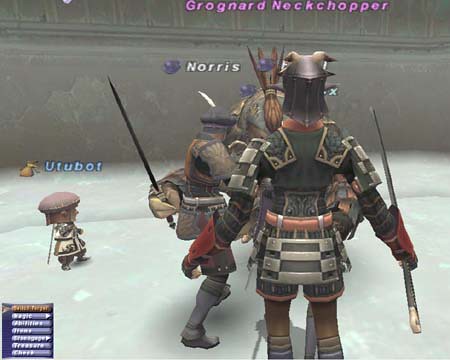This screenshot from a video game features a cast of cartoon animated characters, each with their names displayed above them. At the forefront are characters named Grognard, Nock, Neckchopper, and Purple. To their left, a gray-clad character named Norris stands prominently. Additionally, in the bottom left corner, a shorter character named Utu or Utubot is visible, recognized by their smaller stature. Each character is adorned in detailed samurai armor, complete with swords in hand, indicative of a warrior theme.

They stand on a light gray, smooth ground, which contrasts sharply with the dark gray, heavily cracked walls surrounding the room. The environmental textures emphasize a battle-worn or ancient setting. At the bottom left of the screen, white text accompanies a blue square text box, likely providing game-related information or instructions to the player. This vivid depiction encapsulates a moment within the game, highlighting both the distinct characters and the intricate environment they inhabit.